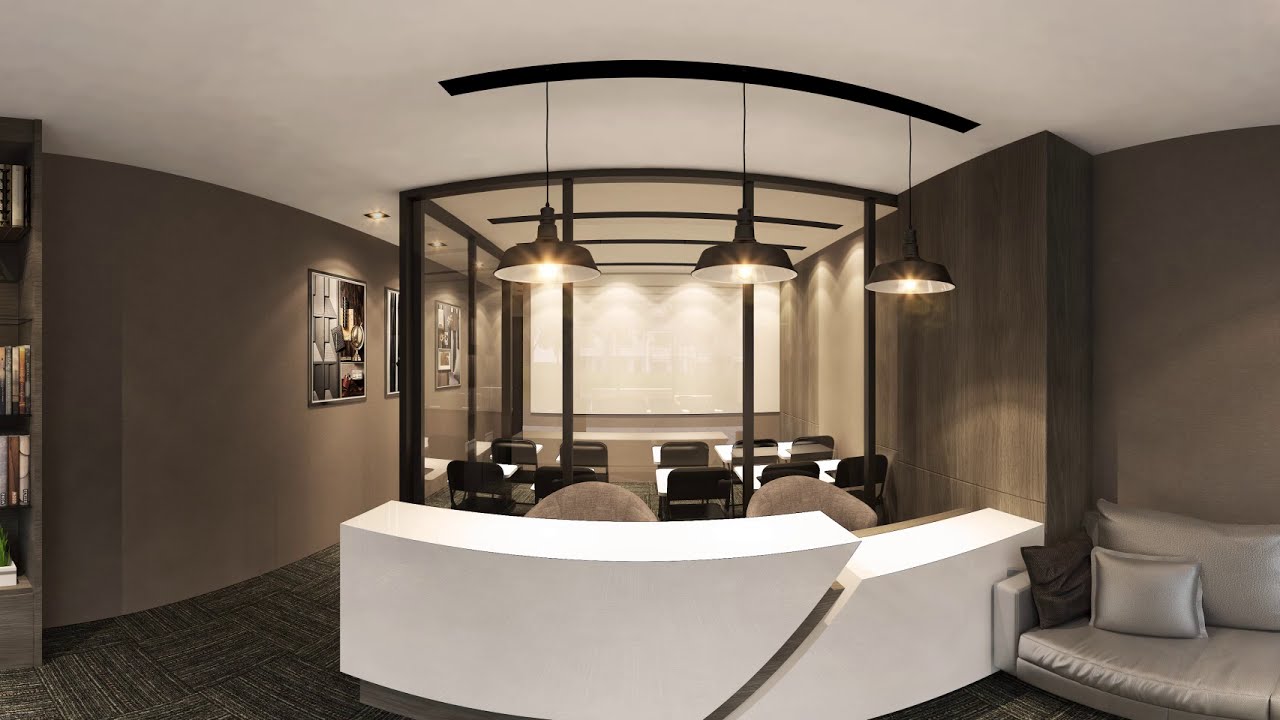This image showcases a beautifully designed conference area captured with a slight fisheye lens perspective. The setting features a mix of modern and stylish elements, all situated indoors. Dominating the center of the image is a long, Art Deco-inspired table with a distinctive diagonal slash cutout, complemented by chairs. Surrounding this central feature, towards the top and sides, are smaller tables with chairs, suggesting a flexible seating arrangement.

The right side of the image hosts a small, cozy sofa adorned with throw pillows. A notable element on the left is a cropped bookshelf that adds a touch of practicality and elegance. Artwork graces the left wall, enhancing the sophisticated atmosphere, while the light brown mauve wall with paneling on the opposite side adds warmth and depth. Overhead, stylish warehouse lamps provide ample lighting, suitable for both home and commercial spaces.

Additional features include a projector screen in the back and a glass-enclosed area designed for presenting, equipped with a screen and a small stage, making the space versatile for various conferencing needs. The flooring is carpeted, contributing to the overall cozy and formal ambiance of this well-appointed room. The color palette includes shades of black, white, gray, and touches of yellow, which tie the elements together harmoniously. There is no text present in the image.